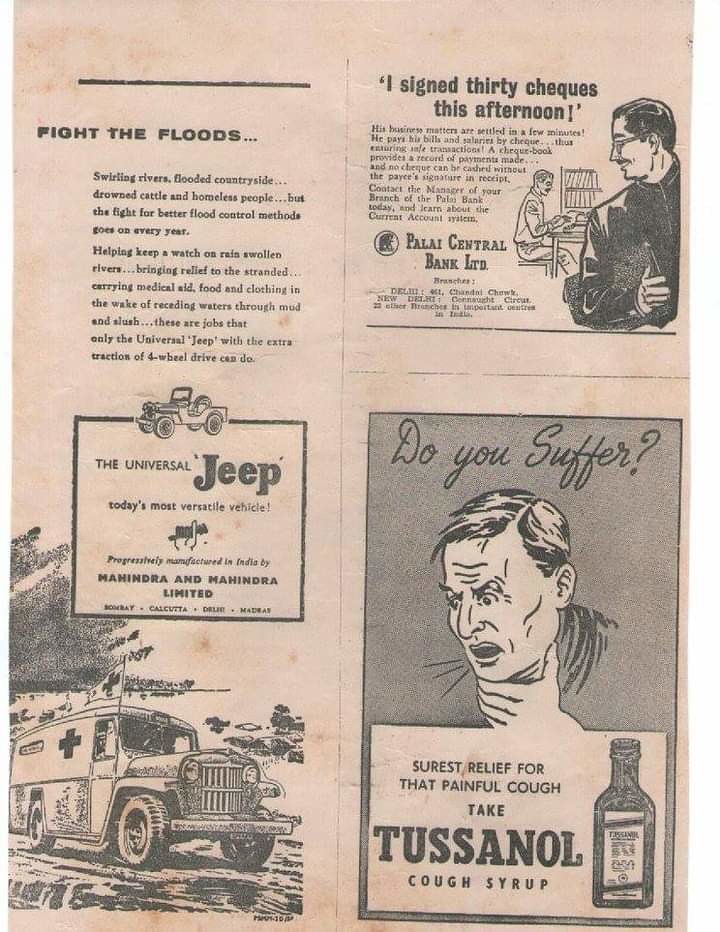This is an old magazine page with a sepia-toned, aged background. The left side features an advertisement for the Universal Jeep, emphasizing its crucial role in flood relief efforts with the bold headline "Fight the Floods." The accompanying text describes how the versatile Jeep, with its four-wheel drive traction, helps monitor rain-swollen rivers, delivers medical aid, food, and clothing, and brings relief to stranded people in flood-hit areas. Below the text is an illustration of a Jeep configured as an ambulance. On the top right, another ad shows a man smiling and walking with a briefcase, captioned, "I signed 30 checks this afternoon," while another man sits at a desk in the background; this promotes the Palai Central Bank. The bottom right corner features an ad for Tuscanol cough syrup, starting with the headline "Do you suffer?" and depicting a man coughing into his hand, offering the remedy as the "surest relief for that painful cough."